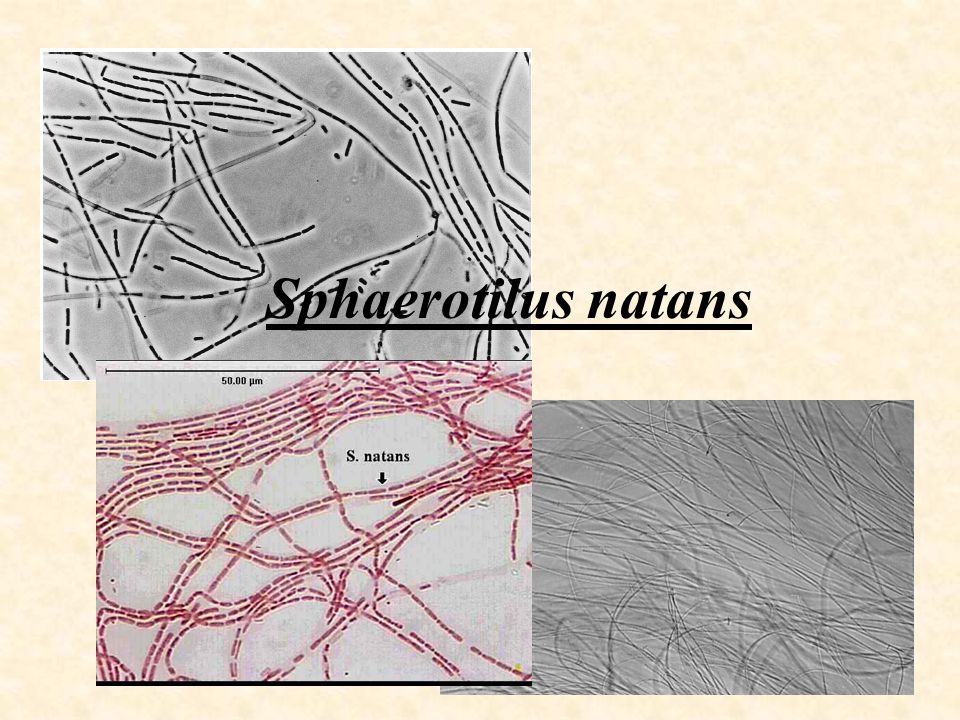This image is an informational slide or graphic in landscape orientation, presenting three distinct pictures related to the Sphyroteles natans, likely a biological component seen through advanced microscopy. Two of the images, positioned on the top left and bottom right, are black-and-white, resembling Scanning Electron Microscope (SEM) or Transmission Electron Microscope (TEM) photographs, displaying highly magnified stringy biological structures against a gray background with random black lines. The third image, placed on the bottom left, is a color-enhanced version of the same type of structure, featuring prominent red strands with an arrow labeled 'S' pointing towards a central red line and a scale bar indicating a range of approximately 50 microns. The entire graphic has a cream-colored parchment texture. Overlying the pictures is a black italic heading with scientific notation reading "SPHYROTELES NATANS," adding a formal scientific touch to the presentation.